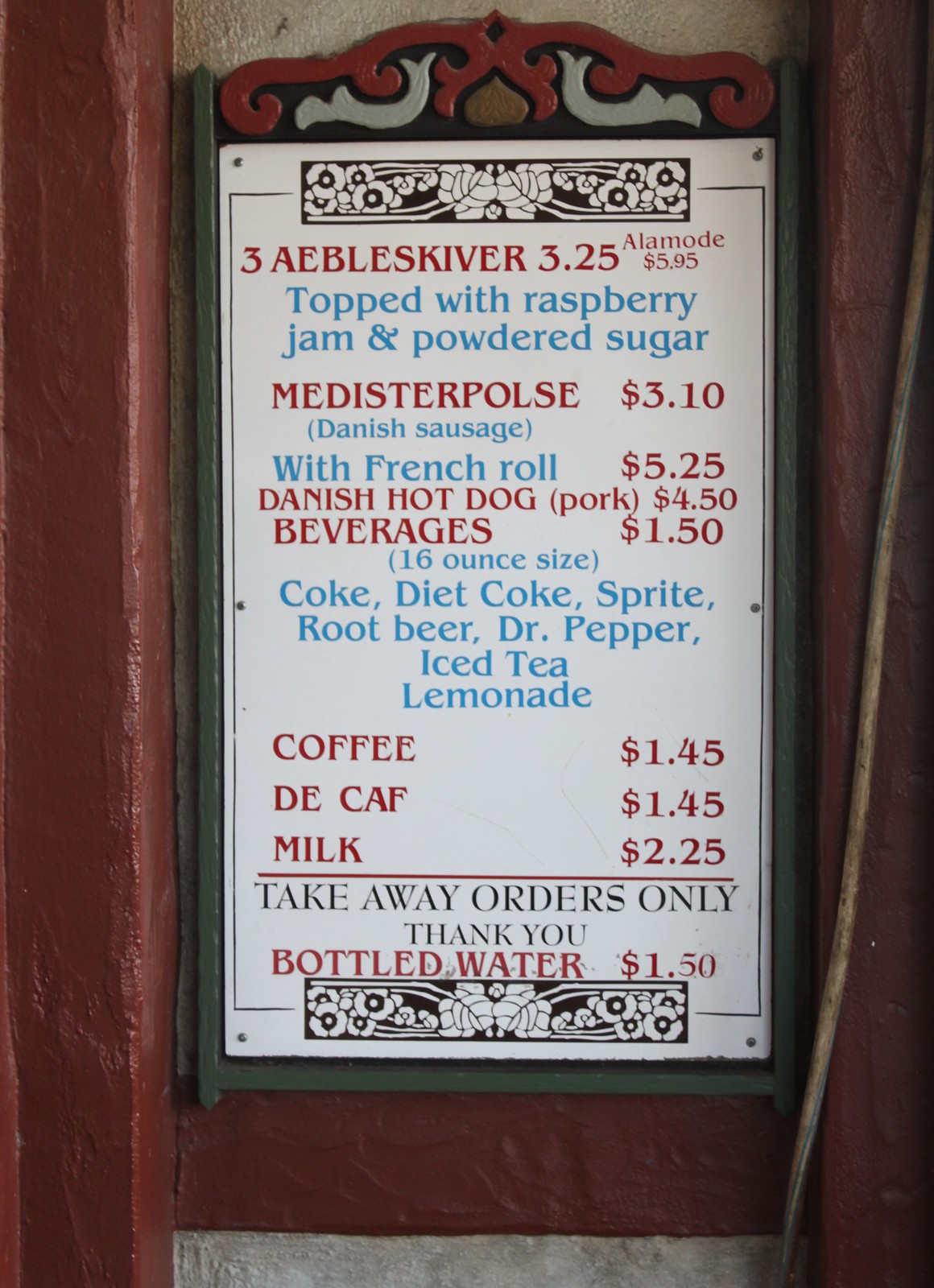This photograph captures an outdoor menu sign for a quaint, atmospheric restaurant. The menu is mounted on a wall adorned with decorative details in dark red and dark green hues, providing a rustic and charming backdrop. The menu itself features a white background with red and blue text, and is topped with an elegant black-and-white floral design, adding a touch of sophistication.

The menu items listed are as follows:
- **Three Able Skeever**: $3.25 (a la mode $5.95), topped with raspberry jam and powdered sugar.
- **Medisterpulse** (Danish sausage): $3.10 (with French roll $5.25).
- **Danish Hot Dog** (pork): $4.50.
- **Beverages**: One 16-ounce size for $1.50, available in the following flavors - Coke, Diet Coke, Sprite, Root Beer, Dr. Pepper, Iced Tea, Lemonade.
- **Coffee**: $1.45.
- **Decaf Coffee**: $1.45.
- **Milk**: $2.25.
- **Bottled Water**: $1.50.

The sign also notes that all orders are take-away only, with a polite "thank you" at the bottom.

Overall, the menu not only details various delectable Danish and American offerings but also evokes a sense of coziness and attention to detail.